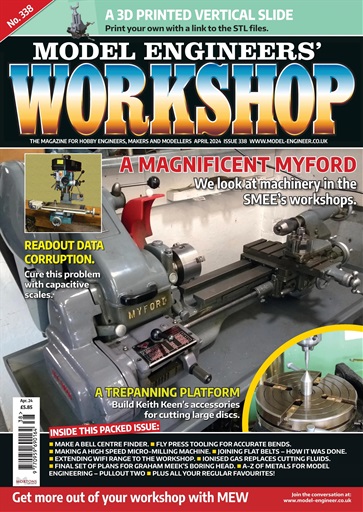The cover of Model Engineers Workshop magazine, Issue No. 338, prominently features a detailed photograph of a gray and black piece of machinery, which appears to be a 3D printed vertical slide. A headline at the top in a green strip invites readers to "Print your own with a link to the STL files." The magazine title, Model Engineers Workshop, stands out in a red triangle in the top left corner.

In the center of the cover, bold text highlights "A magnificent Myford," signaling an in-depth look at machinery in the SMEEs Workshop. To the left, another article title in bold yellow letters reads, "Read Out Data Corruption," with a subtitle explaining how to "Cure this problem with capacitive scales." The bottom of the cover features a red strip that encourages readers to "Get more out of your workshop with MEW." Beneath this, specific projects and tips mentioned include building "a trip panning platform" and Keith Keene’s accessories for cutting large disks.

Additional details for various articles and features inside the issue are listed along the bottom of the cover, alongside the magazine's price, date, and a UPC code for purchasing. The cover is colorful and text-heavy, providing a comprehensive look into the magazine's content.